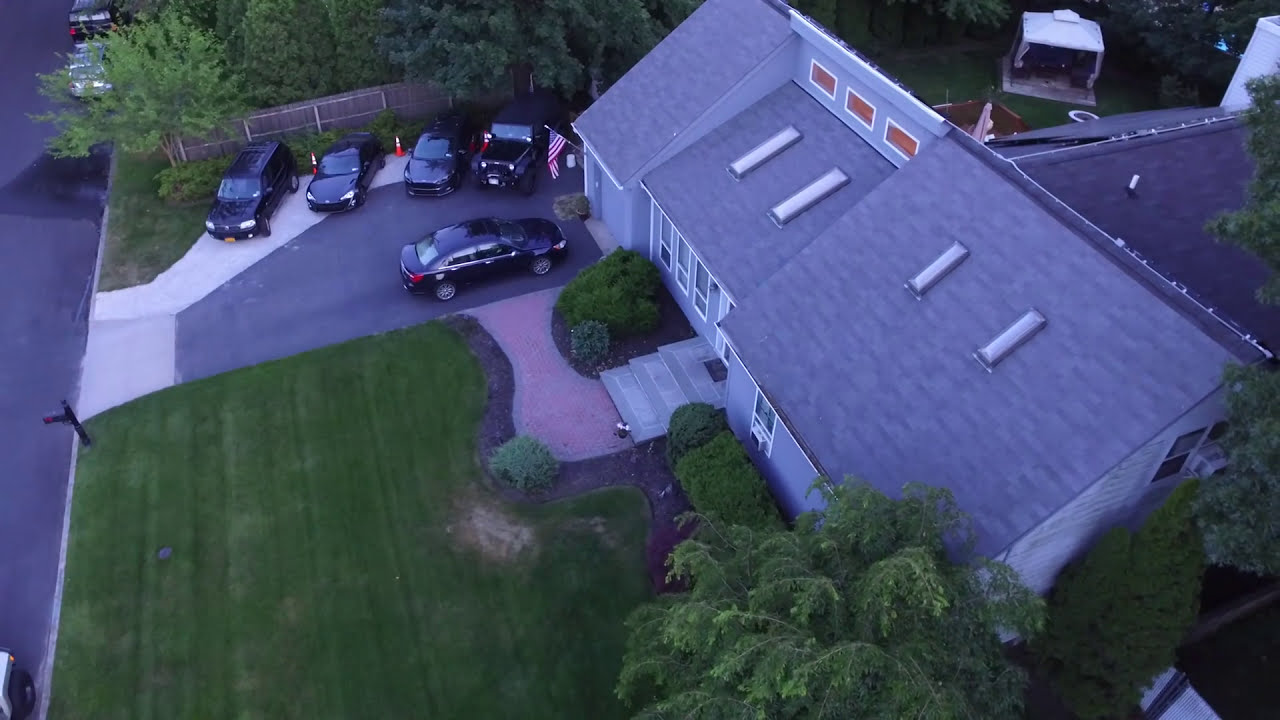The image is a bird's-eye view photograph taken outside during either an overcast day or near night-time, showing a beautifully landscaped house with a greyish-blue exterior and dark grey tiled roofs. The house features four rectangular skylights and extends toward the back. Situated diagonally on the right side, it stands out against the green grassy areas. A paved, pink-colored walkway leads to the house, surrounded by neatly maintained lawns and trees. The driveway, located in front and to the left of the house, hosts five black cars, including a mix of sedans, an SUV, and a Jeep, all parked either parallel or pulled in. Adjacent to the driveway, a paved road runs along the left-hand side of the image.